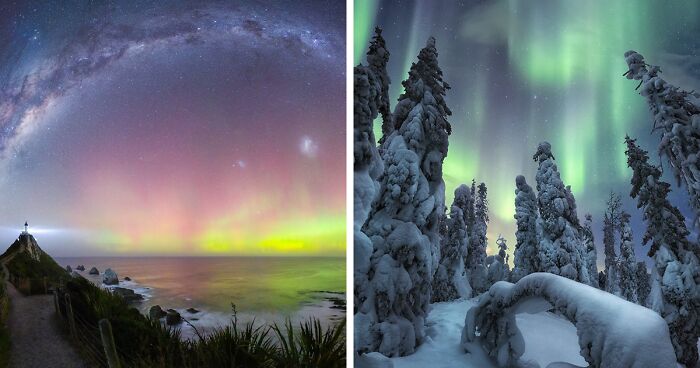The two square-shaped images side-by-side capture the mesmerizing spectacle of the Aurora Borealis in distinct yet equally fantastical landscapes. The left image portrays a serene pathway bordered by a body of water, perhaps the sea or a lake, with a small hill crowned by a lighthouse at the end of the path. The night sky above is an enchanting blend of purplish, pinkish, and yellowish hues, interspersed with stars and celestial formations arcing across the canvas. A noticeable Milky Way presence enhances the surreal atmosphere. Meanwhile, the right image offers an upward view through a snow-covered alpine forest, featuring tall trees that appear almost ethereal against the backdrop of a clear night sky. Dominating this sky is the breathtaking green light associated with the Aurora Borealis, extending to bluish tones, creating a striking contrast with the pristine, snowy landscape below.